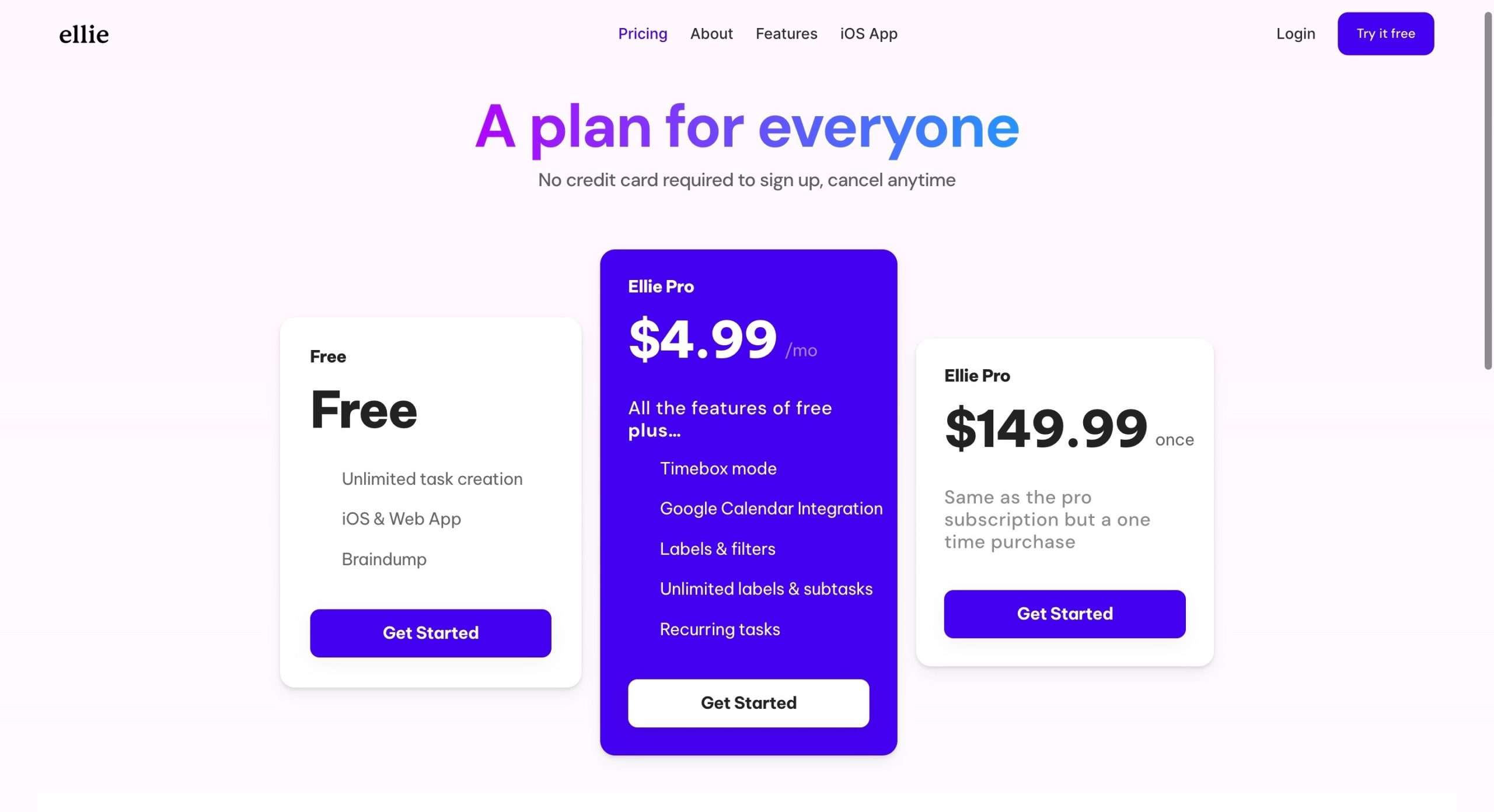Here is a more detailed and cleaner description for the image of the website:

---

The image showcases a website for a platform named "ELLIE." In the upper left corner, the logo "ELLIE" is prominently displayed. 

In the top right corner, options such as "Log Out" and a clickable "Try It for Free" button, highlighted in blue, are visible. The top middle section of the website features navigation links including "Pricing," "About," "Features," and "iOS App."

The central part of the web page prominently displays a welcoming header that reads "A Plan for Everyone." The words "A Plan for" are in purple, while "Everyone" is in blue, with a gradient that lightens as it progresses to the right.

Beneath this main header, there's a note stating "No credit card required," accompanied by "Sign up, cancel any time." 

There are three distinct subscription options prominently detailed in white boxes:

1. **Free Plan**:
   - Title "Free" in bold letters.
   - Offers unlimited task creation across iOS and web apps.
   - Features include "Brain Dump" capability.
   - A "Get Started" button in blue.

2. **ELLI Pro Plan**:
   - Priced at $4.99 per month.
   - Describes itself as including all features of the free plan plus additional functionalities:
      - Time box mode.
      - Google Calendar integration.
      - Labels and Filters.
      - Unlimited labels and subtasks.
      - Recurring tasks.
   - A "Get Started" button in white.

3. **ELLI Pro Lifetime Plan**:
   - One-time purchase priced at $149.99.
   - Offers the same features as the monthly Pro subscription.
   - A "Get Started" button in blue at the bottom of the box.

The overall design uses contrasting colors and a clean layout to help distinguish between different sections and plans.